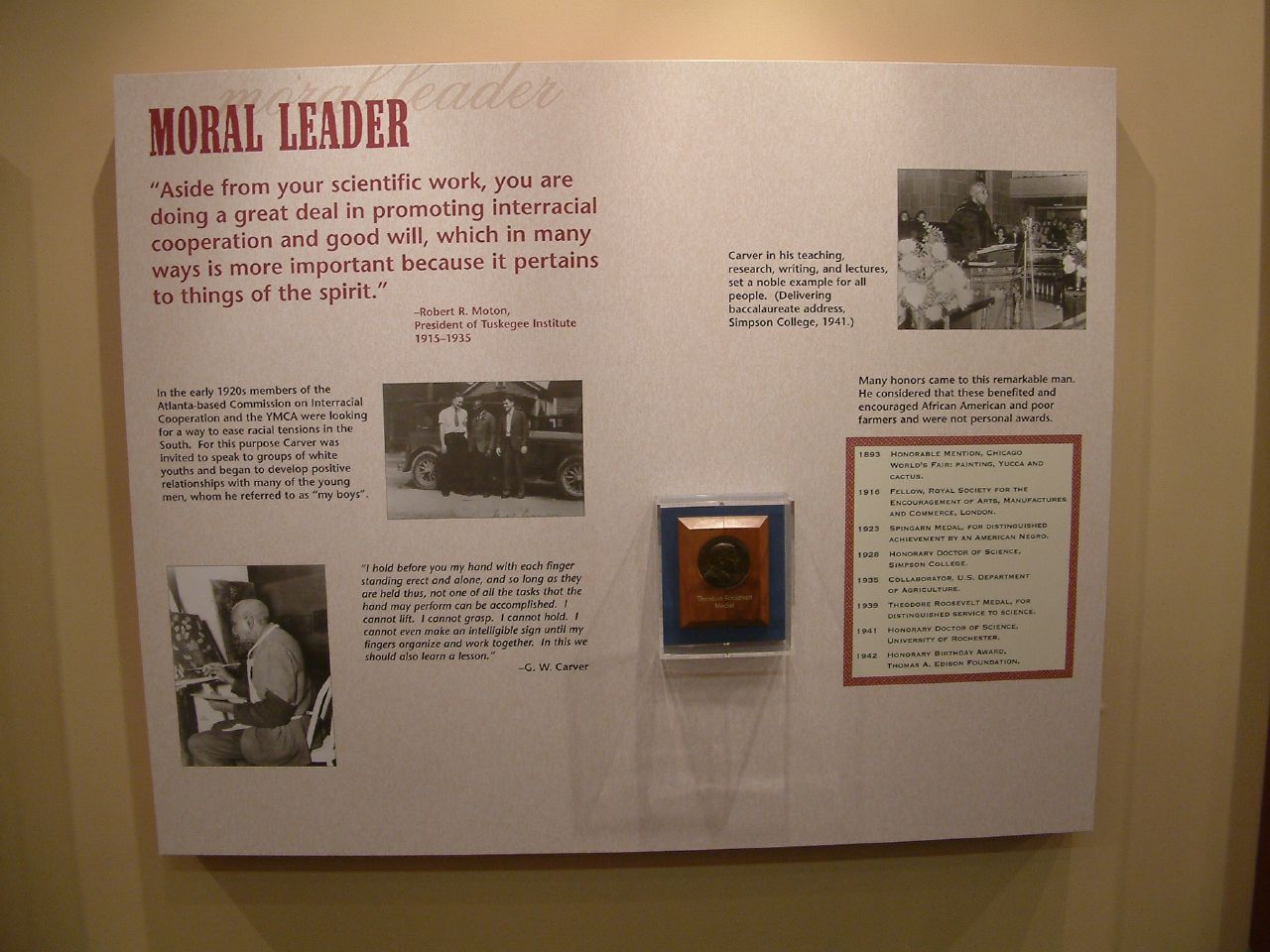This museum placard, mounted on a beige wall, features a white square display adorned with images and text. Prominently at the top left, in large red letters, is the phrase "Moral Leader." Beneath this title is a quote from Robert R. Moton, president of Tuskegee Institute from 1915 to 1935: "Aside from your scientific work, you are doing a great deal in promoting interracial cooperation and goodwill, which in many ways is more important because it pertains to things of the spirit." This central quote sets the theme for the display.

The placard includes several black-and-white photographs. One depicts three men standing in front of an old automobile: the two on the outside appear to be white, while the man in the middle is African American. This photograph is accompanied by text that references the early 1920s and mentions members of the Atlanta-based Commercial of International Cooperation and the YMCA, indicating a historical context for the promotion of interracial activities.

Another photograph shows a man possibly sitting in front of an easel, appearing to draw. Above this image is a black-and-white photo of a man standing behind a podium, addressing a group. There's also a depicted list of years and significant events in a small beige panel on the bottom right of the display. Additionally, the display features a push button in the center, encased in a brown square inside a larger blue square with a white border, potentially an interactive element.

Interestingly, the display might pertain to the George Washington Carver Museum, given that one of the captions discusses Carver's efforts in promoting goodwill among young white men, alongside other informative texts about his teachings and speeches. Central to the exhibit is a coin displayed on a wooden base under glass, signifying its historical value. The placard provides a detailed portrayal of Carver's legacy in fostering interracial cooperation during his time at the Tuskegee Institute.